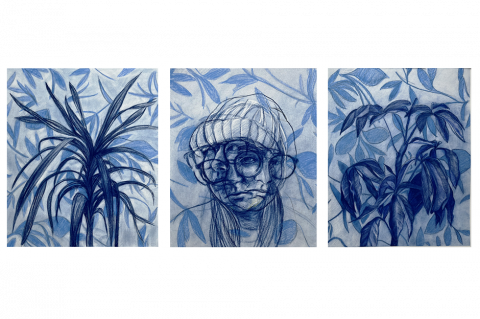This image is a triptych featuring three distinct yet thematically cohesive panels. The left and right panels both showcase artistic renderings of plants in varying shades of blue, white, and dark blue. The plant in the left panel appears spiky, casting intricate blue shadows against a light blue background. Conversely, the plant in the right panel features more rounded leaves but maintains the same color scheme and shadow play. The central panel diverges as it depicts a multi-angled portrait of a serious-looking woman wearing a white beanie and black-rimmed glasses. The woman’s face is fractured into three different expressions, looking left, down-left, and right, creating a surreal, overlapping effect. The plants in the middle panel are relegated to the background, further emphasizing the woman's intense, contemplative gaze and the repetition of her persona in various directions. Together, these panels contrast natural elements with human presence, unified by the consistent use of blues and whites.